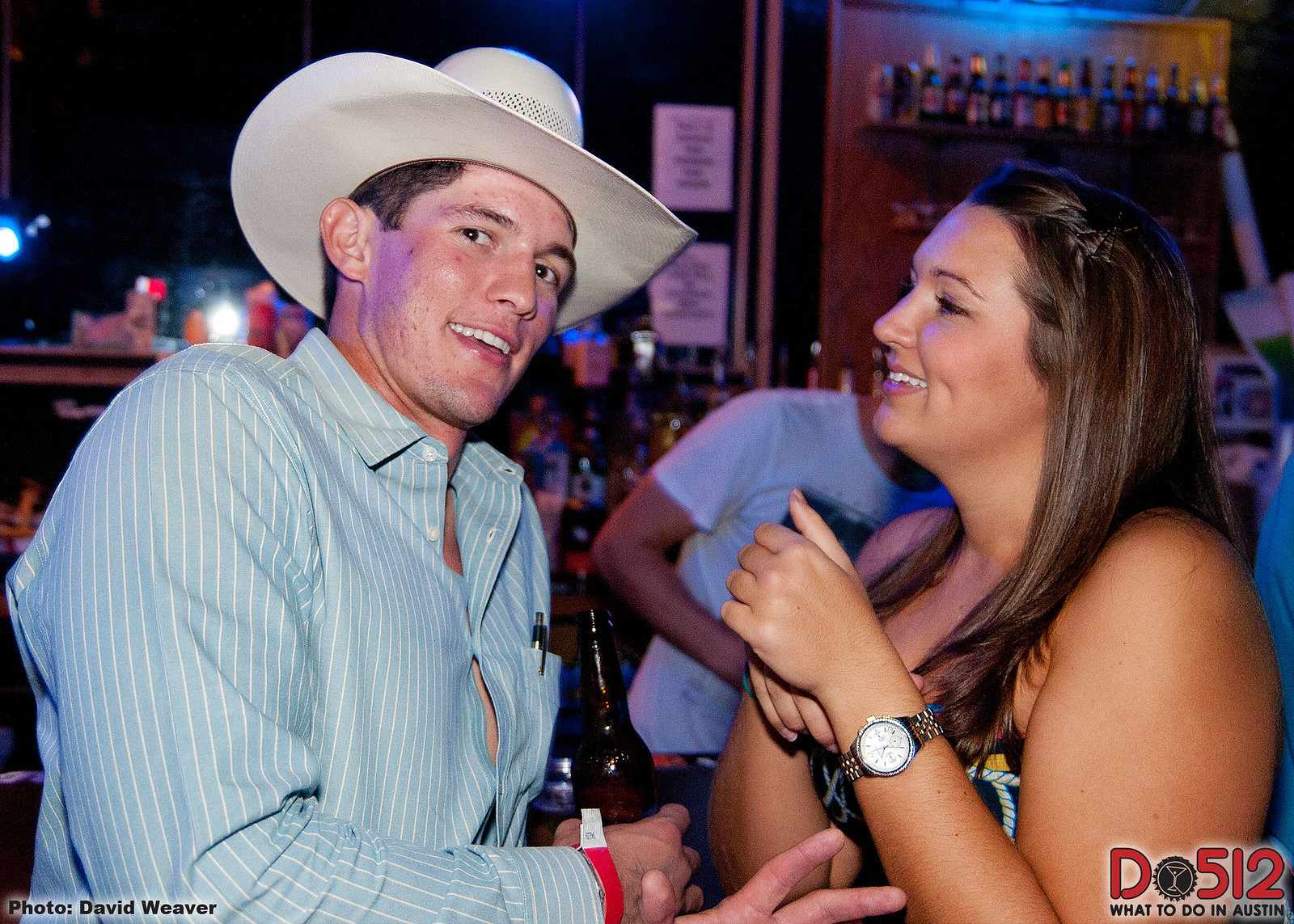In this lively scene set in a bar, a young Caucasian man and woman are captured enjoying their evening, possibly in Austin, Texas. The man on the left, dressed in a light blue collared shirt with white vertical pinstripes and a white cowboy hat, looks directly at the camera. His shirt, slightly open at the top, revealing his skin, and a pen is visible in his left pocket, while a red wristband circles his right wrist. He smilingly holds a bottle of beer in his right hand. The woman beside him, also Caucasian with long dark brown hair cascading over her shoulders, gazes at him affectionately while smiling. She wears a dress with exposed arms and a silver watch on her left wrist, with her right hand holding a glass. Behind them, the bar's shelves showcase a variety of bottles, and a bartender in a white t-shirt leans over the counter. Additional details include the words "Do 517. What to do in Austin?" in the lower right corner, implying the location, and "photo, David Weaver" alongside a martini glass icon and the number "512."